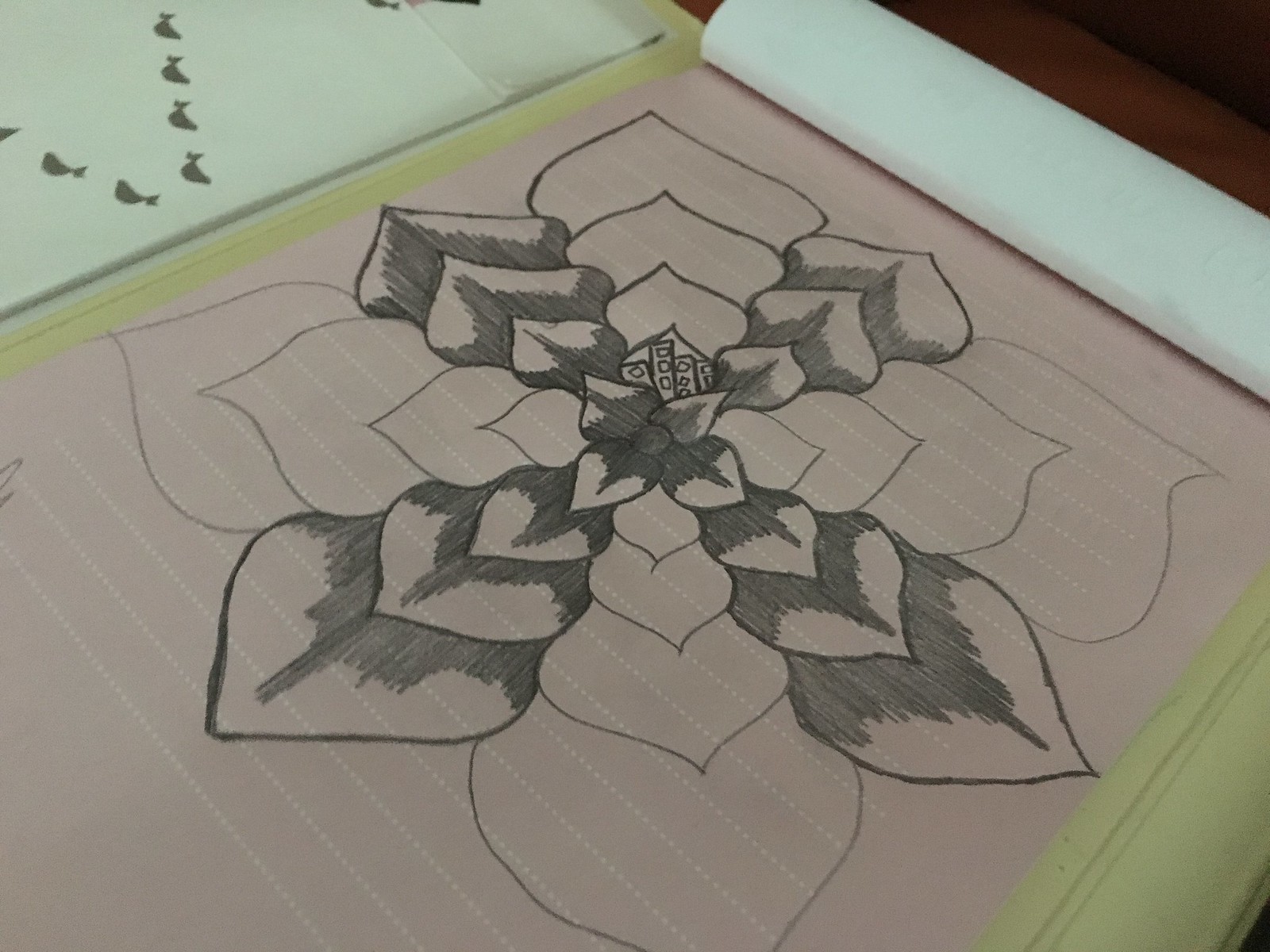This detailed caption describes an artwork in progress:

The image features a close-up of a partially completed drawing set against a pinky-gray paper background. An ivory-toned frame surrounds the artwork, adding a subtle contrast. In the upper right corner, a roll of white paper is visible, possibly containing additional sketches or serving as a tool for the artist.

The drawing itself depicts a meticulously detailed flower bud. It starts with simple lines that form the basic structure of the flower. The flower consists of four concentric layers of petals, with each layer containing eight distinct sections, summing up to a total of eight petals per layer.

At the center of the flower, there is a detailed section likely representing the stigma, surrounded by four prominently outlined petals. Extending beyond this central portion, there are additional sets of petals creating a symmetrical and harmonious design.

The artist has used either charcoal or pencil to shade half of the petals, giving them a rich gray tone that contrasts with the untouched sections still revealing the pinky-gray hue of the paper. Four of the petal sections have already been shaded, while the remaining sections are still in the preliminary stages. One of the sections yet to be fully detailed displays a small petal adorned with tiny rectangles and irregular shapes, hinting at the intricate details to come.

The image beautifully captures the artistic process, showcasing both the raw beginnings and the budding complexity of the flower drawing.